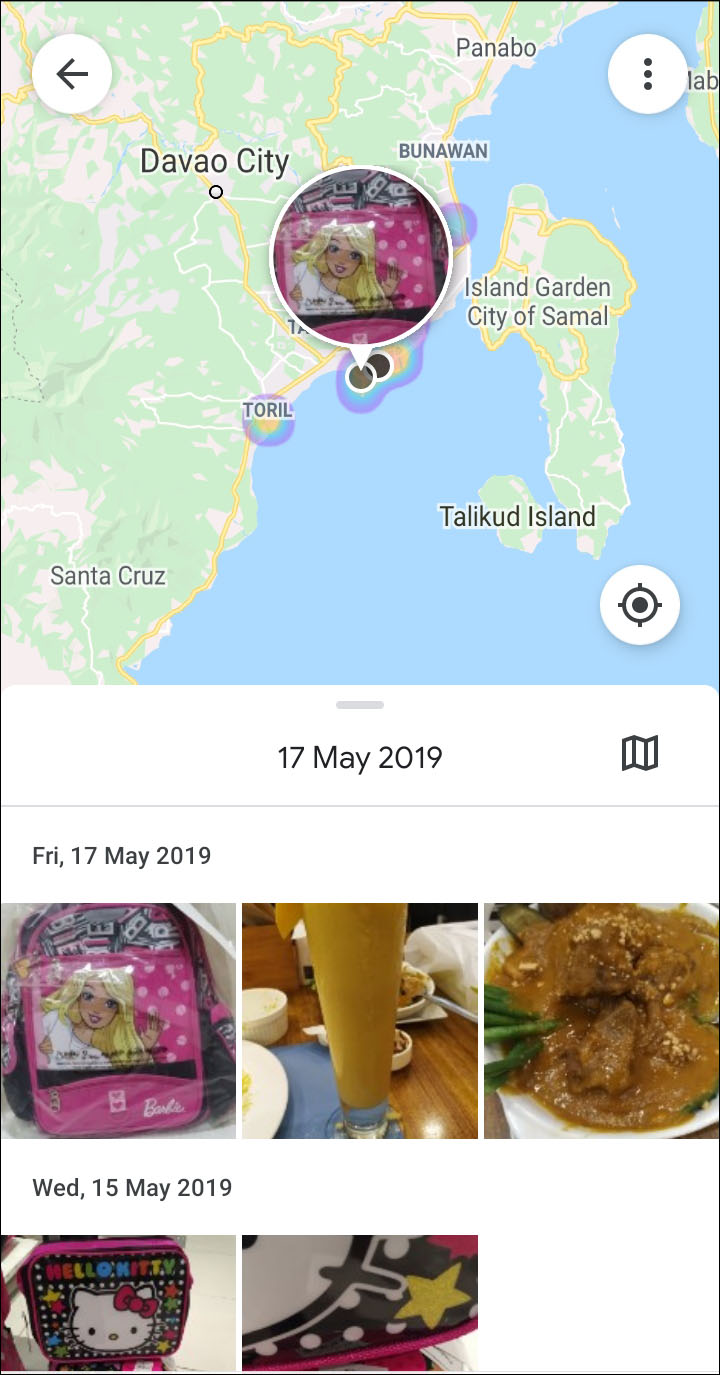This screenshot showcases a map primarily displaying land and water features. The map is divided with sky-blue water stretching from the top right to the lower left, while the remaining land is depicted in light green and beige hues. At the center of the map, there is a circular icon featuring an anime-style character with blonde hair and a white dress. 

On the left side of the map, several cities are marked: Davao City located centrally, with Santa Cruz to its south, and Panabo and Bunawan to its north. To the right, the Island Garden City of Samal is prominently visible, accompanied by a smaller island named Talikud Island just below it. The upper left corner contains a small circle with a left-pointing arrow within it. Below the map, set against a white background, is the date "17 May 2019."